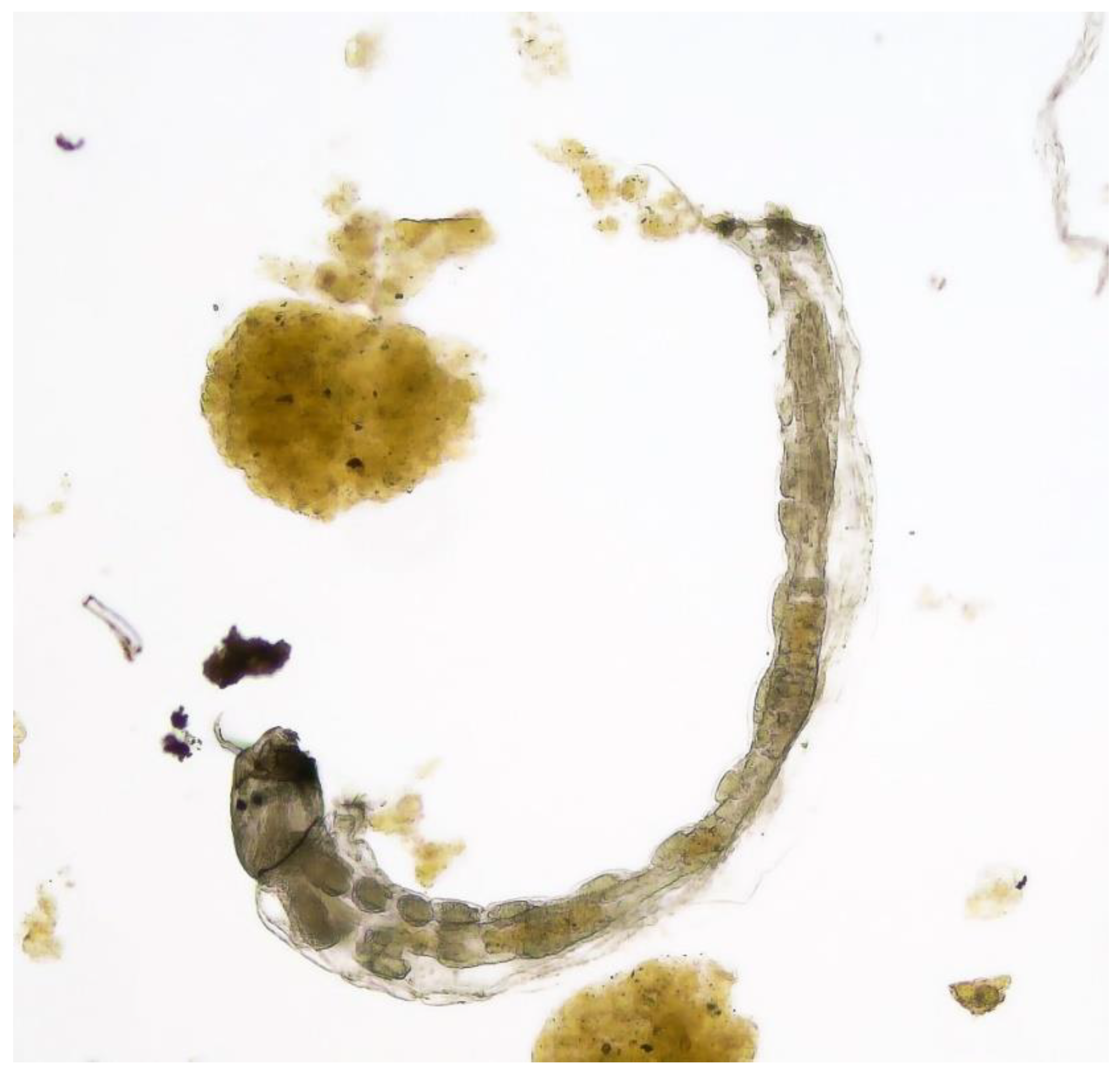The image showcases a detailed view under a microscope, possibly capturing a specimen from medical or biological research. Central to the composition is a long, gray parasite or insect with a distinctly curved tail reminiscent of a "J" shape, which forks upwards towards the left. The insect’s head, situated near the bottom right of the image, features visible eyes and antennae. Surrounding the insect are various dark and greenish specks and blotches, with some green areas suggesting possible viral elements. The backdrop of the slide is a light blue, adding contrast to the grayish and brownish-yellow hues of the insect and its secretions. The overall scene is an intricate mix of biological components, hinting at a meticulous study of the specimen's internal and external attributes.